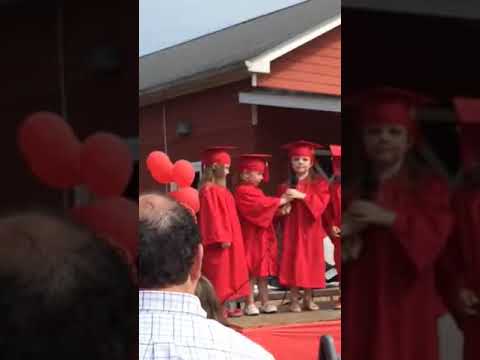This photograph captures a poignant moment from a kindergarten graduation ceremony held outdoors on a pleasant day. At the center of the image are three little girls, around the age of five or six, dressed in red graduation caps and gowns. One of the girls is looking directly at the camera while holding onto another girl, emphasizing their close bond. The focal point remains these three girls, who appear to be in line to receive their diplomas. In the background, there's an orangish-red building with a green awning and a black and white roof, likely part of the school facilities. Adding a touch of festivity, three balloons—one of them distinctly orangish-red—can be seen near the children. In the lower left-hand corner of the image, an older man with black hair and a prominent bald spot, dressed in a white striped plaid scrub shirt, watches the children, probably one of the fathers. The sky is clear, suggesting a perfect day for such a special occasion. This image encapsulates a small, intimate section of the graduation, focusing on the innocence and excitement of the young graduates.